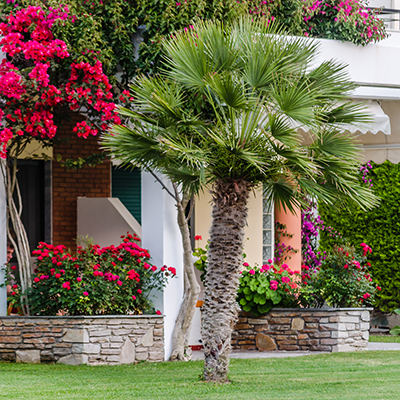The image is a vibrant color photograph of a meticulously maintained, lush green lawn with a central, healthy palm tree characterized by its multiple green leaves. The setting features stone planters on either side of the palm tree, teeming with a variety of bright red and pink flowers and lush greenery. Behind the planters, additional tall flowering bushes can be seen. The backdrop includes a white structure with some brown elements, likely a house, with a red brick facade and green awnings. A white wall and a pillar are also visible, supporting the roof of the building. The landscape is further tied together by the striking contrast of vivid greens and reds of the vegetation, adding to the overall beauty of the image. No people, animals, writing, or motorized vehicles are present in the photograph. Hanging greenery is also noticeable at the top of the image, providing a finishing touch to this serene outdoor scene.